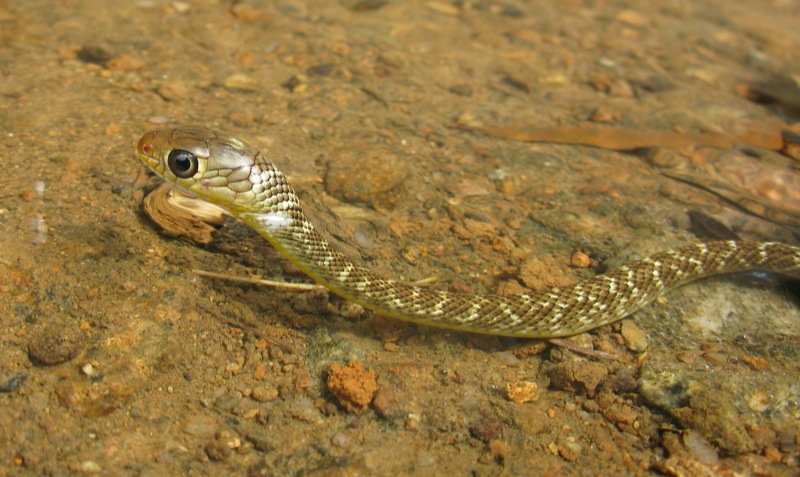In the image, a small snake is slithering through a terrain that appears to be a mix of wet dirt and rocky ground. The snake has a distinctive appearance with a gold-brown body accented by bands of white on its scales, and it blends seamlessly into the natural setting. Its large head, resembling a light bulb, is adorned with a single visible eye that seems to express displeasure. The eye has a dark pupil surrounded by white. The background is a mix of brown dirt and rocks with hues of orange, red, and gray, giving the scene a rich, earthy texture. The dirt looks packed and slightly moist, contributing to the diverse coloration. The snake's body curves slightly as it moves from right to left across the image, with about three-quarters of its length visible, the tail not included. The light reflecting off its scales gives the snake a shiny appearance, further highlighting its young and vibrant nature.